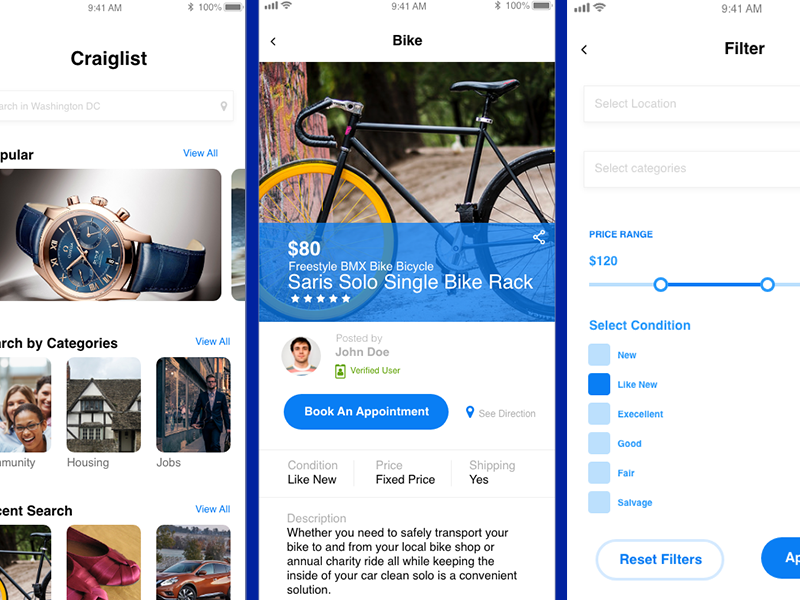This screenshot from Craigslist prominently features the Craigslist logo on the left-hand side in black letters. At the top of the page, three distinct columns are displayed. 

In the first column, the Craigslist logo is repeated directly below, followed by an image of a wristwatch. The watch has a blue face, a blue leather band, and a gold-toned case, with the brand name "Pular" written above it. To the right of the watch, a "View All" option is available. Below this watch, there are additional images, though the text is partially obscured and only shows the letters "RCH." A categorically labeled section titled "View All" is also present.

Underneath this section, the first image features three individuals: a black woman, a white woman, and another person who appears to be a white woman, all smiling. The text beneath this photo reads "Immunity" instead of "Community." Next, there is an image of a Tudor-style house labeled "Housing," followed by a picture of a man in a blue business suit walking down the street, under which the caption "Jobs" is displayed.

In the second column, the word "Bike" is highlighted above an image of a 10-speed bicycle. The bicycle has curved handlebars pointing towards the back and a black seat. At the bottom of this image, there is a banner with the listing: "$80 Freestyle BMX Bike Bicycle, Sarah's Solo Single Bike Rack," along with a five-star rating.

The final column features a section titled "Filter" in black letters. Below it, in blue letters, it states "Price Range: $120," with a slider that users can adjust back and forth.